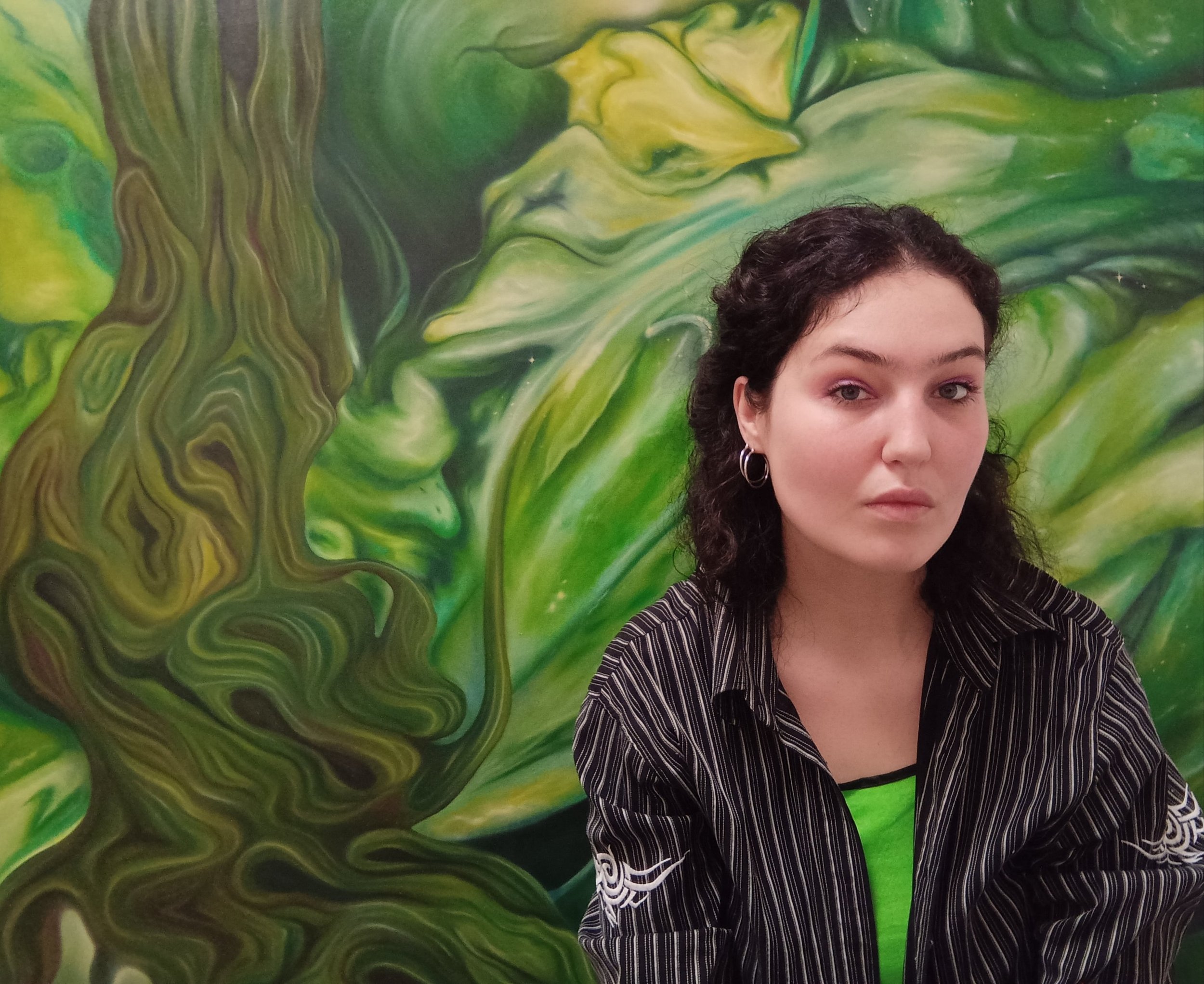The photograph features a young woman positioned on the right-hand side of the image. She is gazing directly at the camera with a serious expression, her eyebrows slightly raised and her eyes half-closed. Her head is cocked slightly to the right, revealing her right ear adorned with medium-sized silver hoop earrings. She has shoulder-length, curly hair that is either very dark brown or black.

The woman is dressed in a black jacket with white vertical stripes and some insignias or emblems on the upper arms. Underneath her jacket, she wears a bright green top. The background is a large, abstract painting dominated by various shades of green, accompanied by splashes of white, yellow, and brown. The artwork behind her evokes an organic, plant-like quality with wavy lines and shapes that could suggest vines, leaves, or a waterfall. The overall composition suggests the photograph might be used for a publicity shot or a social media profile.